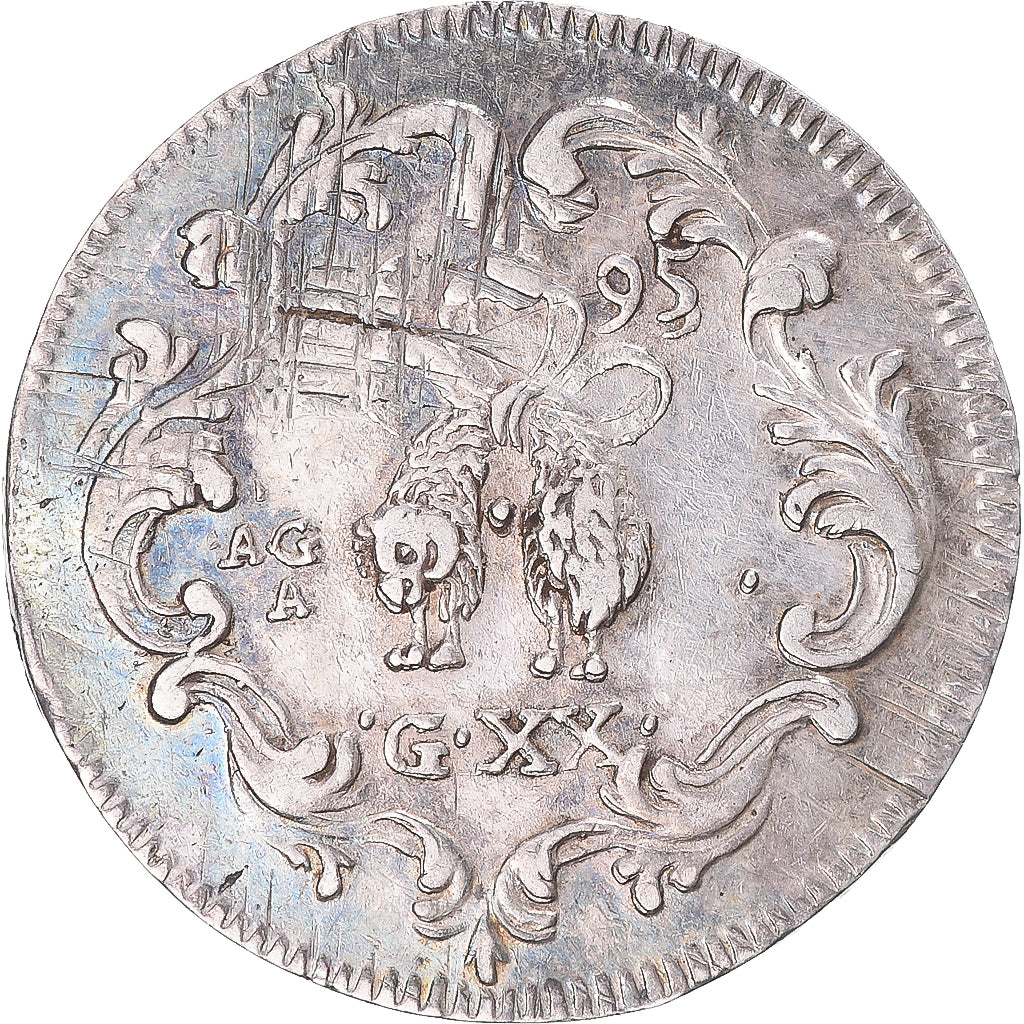This close-up photograph showcases an ancient, weathered silver coin, likely from medieval Europe or earlier. The coin, larger than a quarter, exhibits significant wear and features intricate detailing. The circumference is adorned with scalloped and serrated edges, resembling the pattern one might see when using a fork to press down on ravioli, creating a florally intricate, leafy filigree border. The coin's surface is not smooth, suggesting it was individually hand-stamped rather than mass-produced, adding to its unique, rustic appeal.

At the top right of the coin, the number "95" is prominently displayed, its digits worn but still discernible. Below, on the left, the letters "AGA" are etched into the silver. Dominating the coin's center are two four-legged creatures, likely lions or goats, though their exact species is hard to ascertain due to the coin's age and wear. These animals appear to be standing or interacting with each other. Beneath them, the text "G.XX" is clearly visible.

Noteworthy is the varying coloration on the coin; parts of it exhibit a bluish tinge on the left side and a pinkish hue on the right, enhancing its historical charm. Overall, the coin is a fascinating relic, showcasing the artistry and coinage practices of its time.